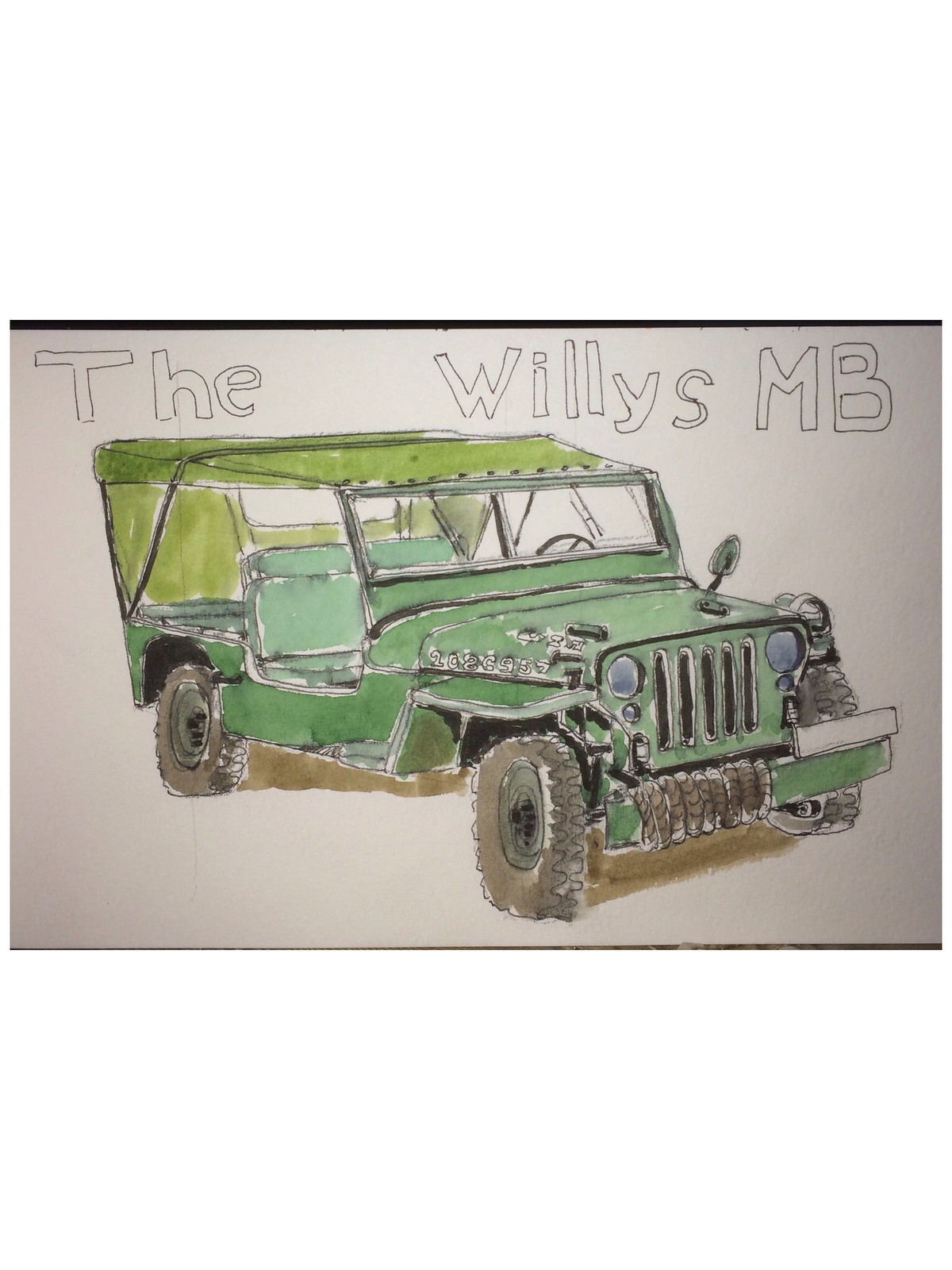The image displays a detailed sketch of a green Jeep vehicle, reminiscent of a Willys MB or a Land Rover-type commonly used by the army. The sketch is on a white rectangular piece of drawing paper, set against a background with a black thin strip at the top and bottom, along with a beige section on the bottom right. Bold, black-outlined text at the top reads "The Willys MB" in bubble or box block letters. 

The Jeep is angled diagonally, with the rear at the upper left and the front at the lower right. Its body is primarily green, featuring a canvas top over the rear section, which is slightly brownish-green, and an open window. The vehicle has no doors on the left side, exposing green benches inside. It is equipped with four large, black wheels, a rope on the front bumper, a single front mirror, and some black strips around the bonnet and trim. The detailed depiction suggests riveted sections and a shallow area for entry. The Jeep appears to be sitting on a dirt ground in the sketch.